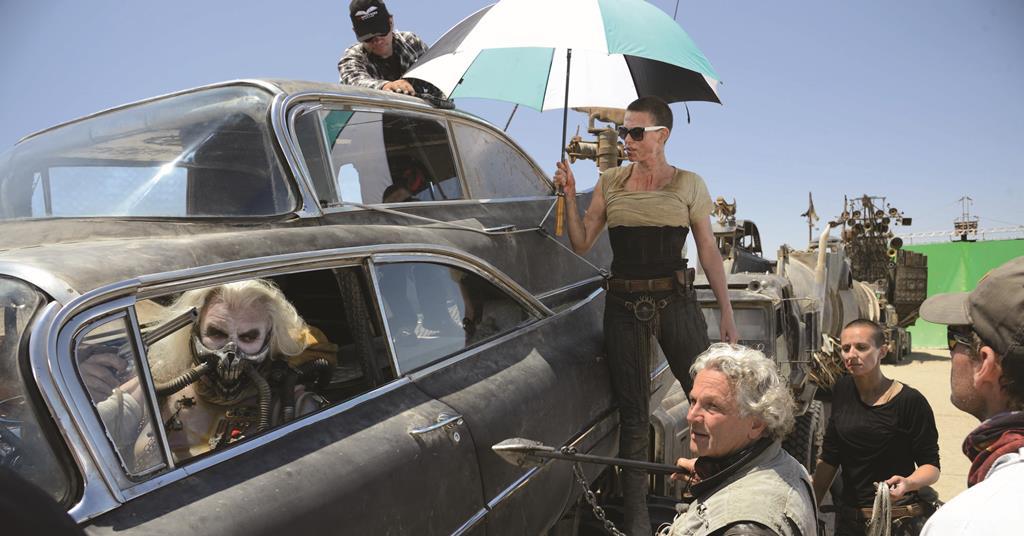The image captures a dynamic behind-the-scenes moment from the set of the movie "Furiosa." It centers on a dusty, old black hearse, positioned diagonally towards the bottom right of the frame. The main antagonist, with long silver hair, is at the wheel, his face obscured by an intricate skeleton gas mask with two prominent air pipes. He is dramatically leaning out the window, brandishing a silver six-shot revolver with his right hand. To the rear of the hearse, a production worker in flannel with a black hat can be seen adjusting something on the vehicle. Beside the car stands a woman with short shaved hair, dressed in black jeans, a black shirt, and a beige crop top, shading herself with a yellow and green umbrella. Surrounding the scene are multiple production crew members, some in costume and some not, with a camera rig positioned in the background. The chaotic, post-apocalyptic aesthetic of the vehicles and characters echoes the thematic elements of the "Mad Max: Fury Road" universe, further emphasized by a procession of similarly grimy trucks and cars filling the backdrop.